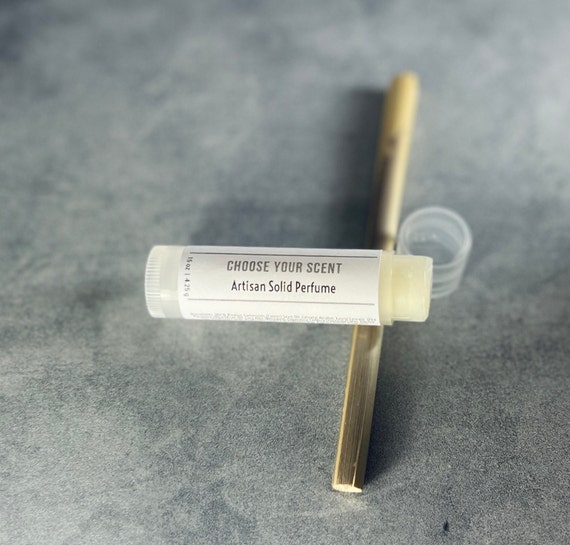This photograph displays an artisan solid perfume container prominently positioned on a smooth, light gray, possibly wood-textured, surface. The container, resembling a lip balm holder, has a white wrap with the inscription "Choose Your Scent" in grey, and "Artisan Solid Perfume" in black. The clear, cap-less capsule reveals a creamy white, balm-like substance at the tip, resembling chapstick. Nearby, the clear plastic cap lies next to a vertical stick-like object, possibly a pen or pencil, creating a T-shape with the horizontal perfume holder. The scene hints at an advertisement setup, showcasing the aesthetically pleasing simplicity of the product.